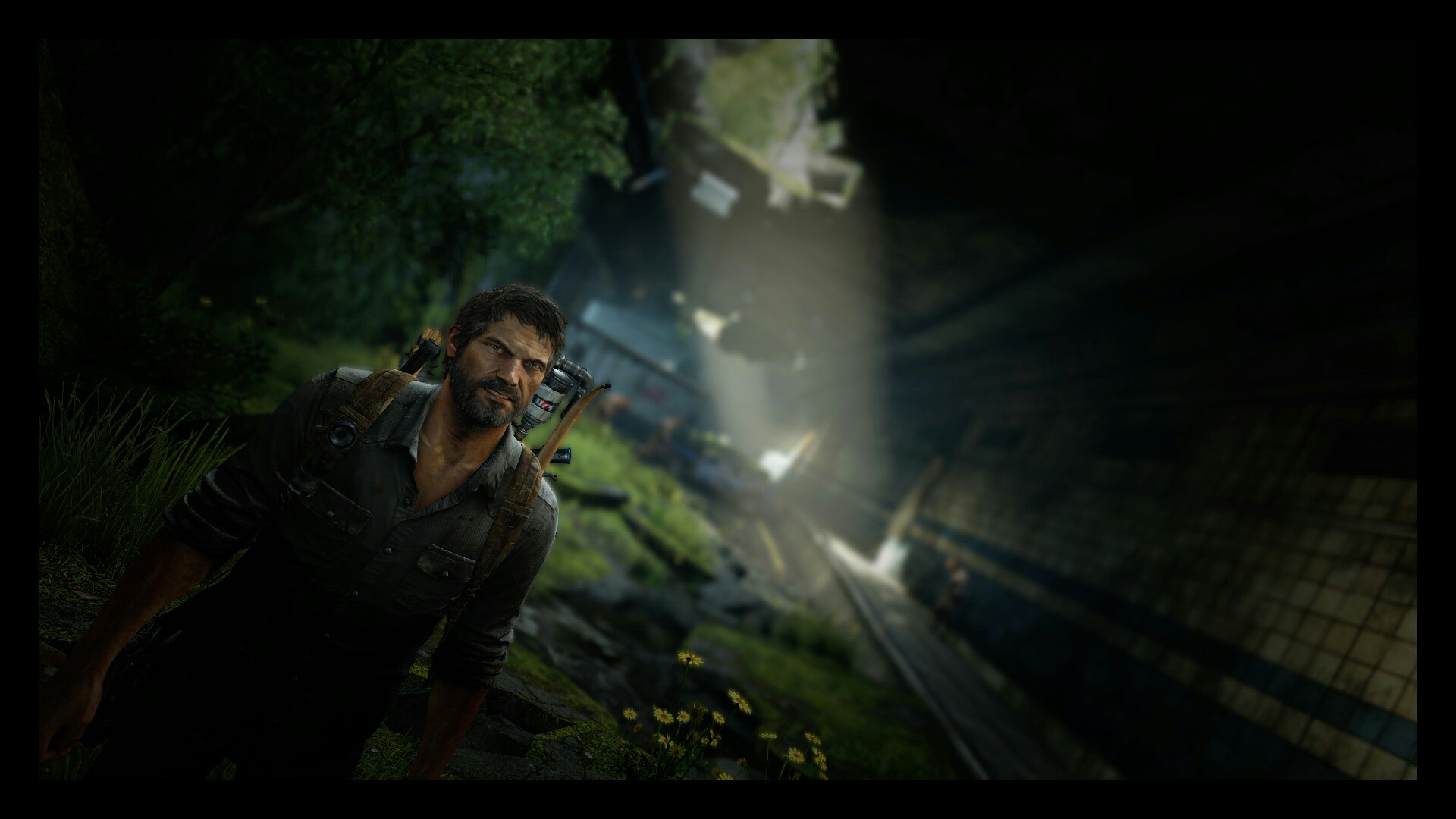The image depicts a rugged man with a dark mustache and beard, accentuated by his piercing scowl. His dark hair is slightly tousled, adding to his intense demeanor. Clad in a long-sleeve shirt, the man appears to be a soldier or perhaps a video game character, given his slightly unreal appearance. Most of his figure is shrouded in shadow, creating an aura of mystery. Affixed to his back is an unidentified object, which does not resemble a traditional backpack. The backdrop is enveloped in darkness, save for a metallic structure partially illuminated by a beam of light descending from above, which casts a dramatic spotlight on the central figure. The overall scene is moody and intense, with an air of tension and uncertainty.